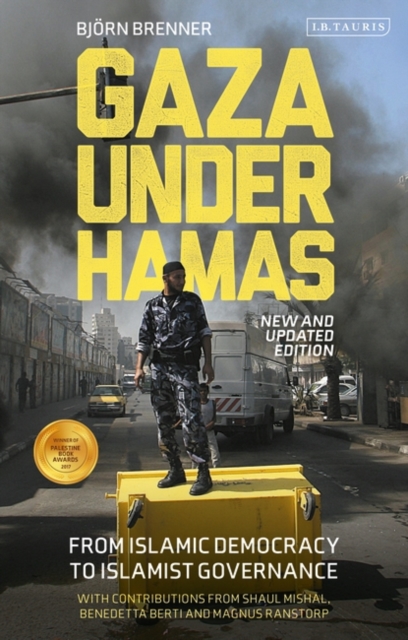The image is a rectangular, portrait-oriented book cover measuring approximately five inches tall and three inches wide. Dominated by a color photograph, the cover features a wartime street scene with buildings on both sides and black smoke billowing into the blue sky. At the forefront, a soldier in gray and black camouflage and black boots stands atop an overturned yellow dumpster. The soldier appears to be of Middle Eastern descent and his head partially obscures the bold, large yellow text which reads "Gaza under Hamas."

The top of the cover features author names in white text: "Bjorn Brenner" positioned left of center, and "I.B. Taurus" in a white rectangular outline to the right. Just below the headline, in small white text, are the words "New and Updated Edition." At the very bottom of the cover, in white text, is the subtitle "From Islamic Democracy to Islamist Governance," with a round gold medallion or emblem positioned near this text. Beneath the subtitle, in yellow text, it reads "With contributions from Shaul Mishal, Benedetta Berti, and Magnus Randstorp." The overall design integrates typography and graphic elements with color photography, underscoring the book's thematic focus.